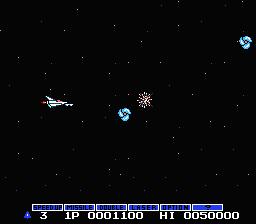This image depicts a screenshot from an old video game, presented in a small, square format. Set against a black background with numerous scattered white dots, the scene likely represents outer space or a night sky. Positioned towards the left center of the image is a white spaceship, appearing to move from left to right. A trail of orange flame extends from its rear, simulating ignition and forward momentum. 

In the center of the screen, there is a round, bluish-gray object, accompanied above by what looks like a firework-like formation. Both objects are relatively small, slightly smaller than the spaceship itself. Another bluish-gray object is located in the upper right-hand corner of the image.

At the bottom of the screen, there are several blue bars containing text labels such as "Speed Up," "Missile," "Double," "Laser," "Option," and a question mark, accompanied by some numerical values. This part of the interface seems to represent various game options or power-ups available to the player. Overall, the image captures the vintage aesthetic and gameplay elements typical of early space-themed video games.